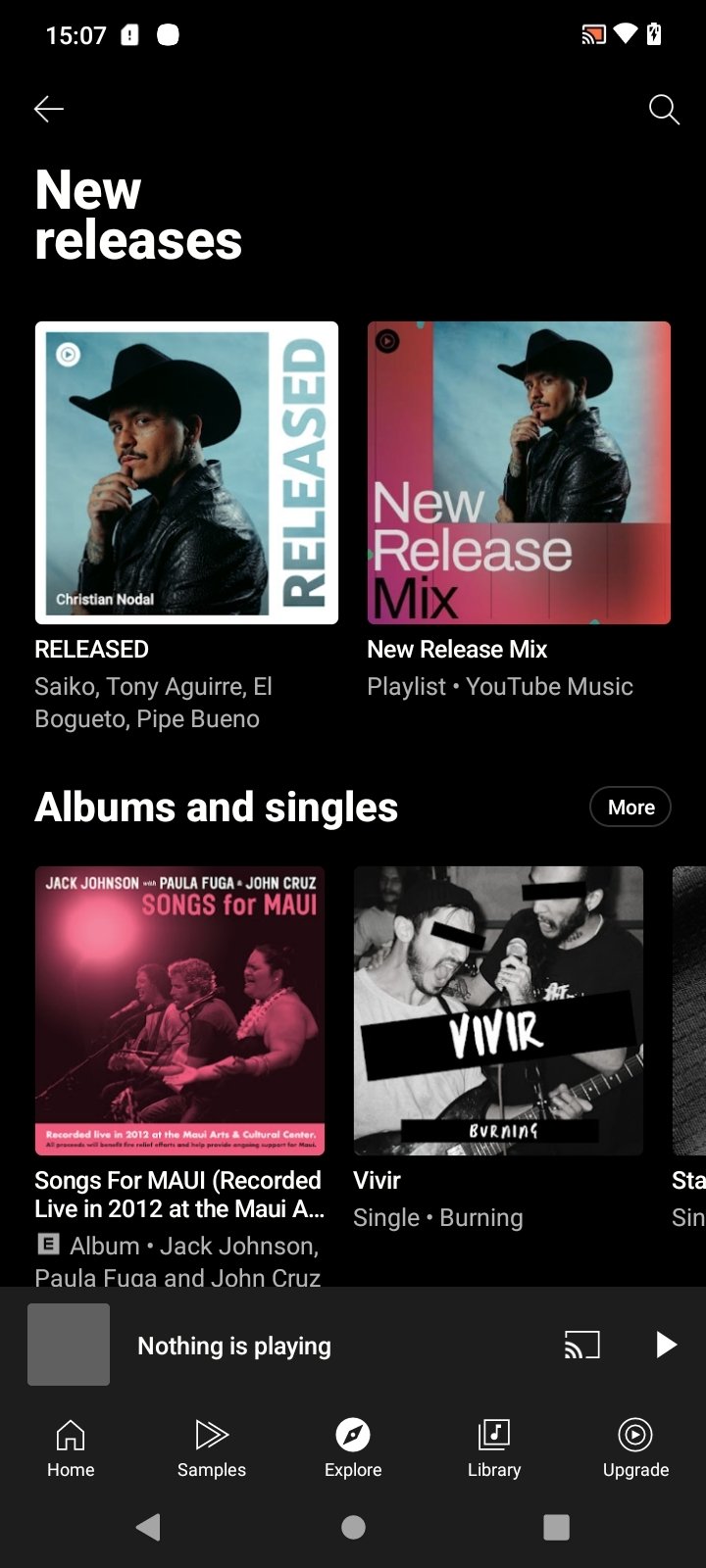Here is the cleaned-up and detailed caption:

---
This image is a screenshot of a mobile device, either a smartphone or tablet, with a black background. The time displayed at the top of the screen is 15:07. The top bar of the screen features various white icons, including a charging battery indicator, Wi-Fi signal strength, a screen-sharing icon, a search icon represented by a magnifying glass, and a back arrow.

The main focus of the screenshot is the YouTube Music player interface, specifically the 'New Releases' section. Two albums are visible within this section. Highlighted is an album featuring an artist in an all-black ensemble, comprising a black leather jacket and a black cowboy hat, by Christian Nodal. Additionally, categories for 'Albums' and 'Singles' are present. One entry in these categories is titled "Song from Maui," recorded live in 2012, although part of the title appears unreadable.

At the bottom of the screen, five navigation buttons are visible: 'Home,' 'Samples,' 'Explore,' 'Library,' and 'Upgrade.'
---

This caption gives a comprehensive description of the elements present in the screenshot.